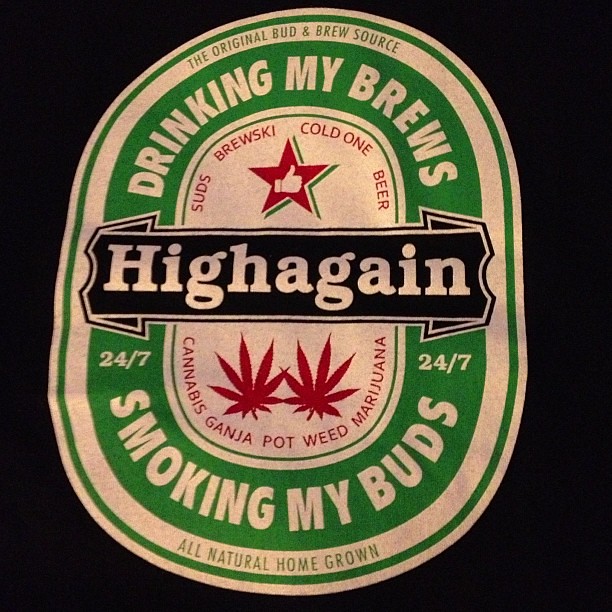This image depicts a logo that parodies the iconic Heineken beer symbol. Against a black background, there is an oval-shaped emblem with a thick outer green circle enclosing a white inner circle. At the very center of this white circle is another smaller white circle. Inside the small white circle, the top features words such as "suds," "brewski," "cold one," and "beer," while the bottom includes "cannabis," "ganja," "pot," "weed," and "marijuana." 

A red star with a white thumbs-up symbol adorns the top of the logo. Across the center, on a black horizontal label within the white circle, the words "High Again" are prominently displayed flanked by "24-7" on either side. Below this, there is the phrase "smoking my buds" with two green marijuana leaves at the bottom. Additionally, the phrase "Drinking my brews" is also mentioned, hinting that this logo represents an all-natural, homegrown source for both alcohol and cannabis. Colors used in this design are predominantly black, white, green, and red.